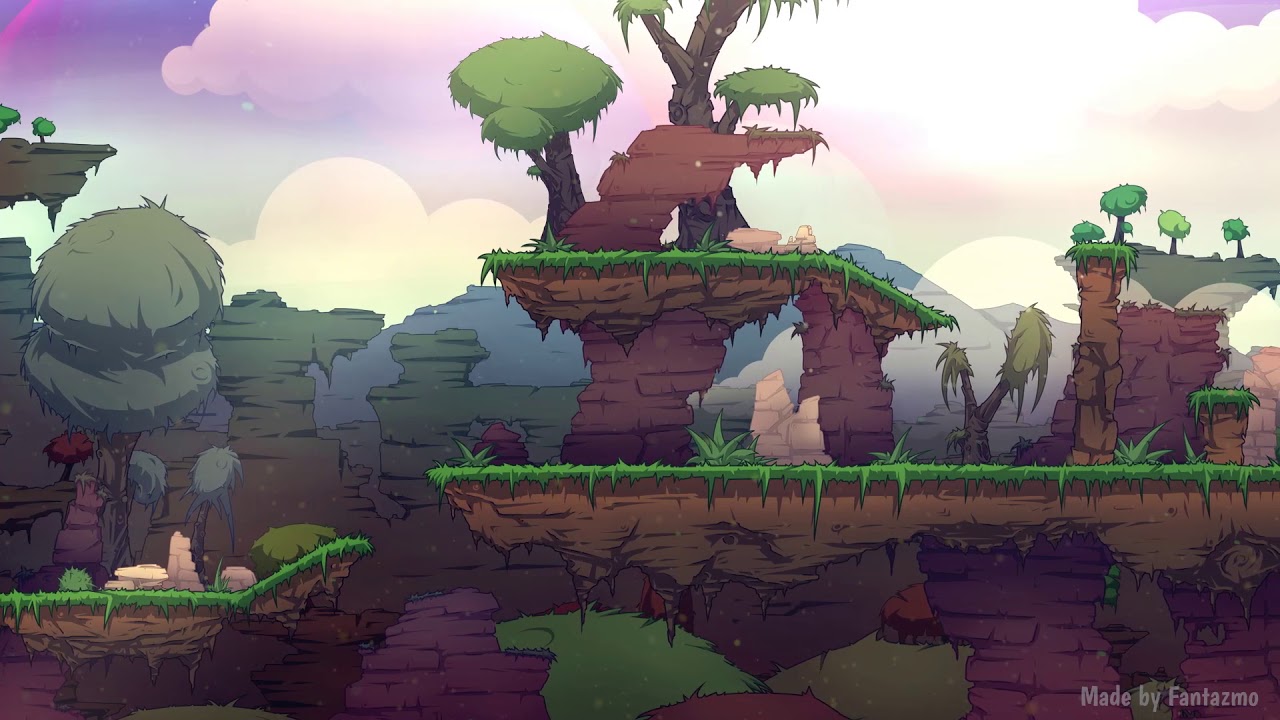This image appears to be a still from an animated or hand-drawn video game background, specifically resembling a 2D side-scrolling platformer. The scene features multiple floating ground platforms at various elevations, creating different levels that a game character could navigate by jumping between them. Each platform predominantly consists of grass and dirt, with some platforms connected by ramps.

Prominently displayed in the bottom right corner is a faint white font that says, "Made by Phantasmo." The background sets a fantasy or sci-fi ambiance with unusual vegetation and a striking purple sky dotted with white clouds. Various natural elements like ferns, plants, bushes, and trees populate the platforms and surrounding landscape. Rocks and mountains are also visible, adding to the rugged, otherworldly terrain. The overall color palette includes greens, purples, and browns, enhancing the whimsical and fantasy-like atmosphere. There are no people present in the image, emphasizing the serene and mystical environment.